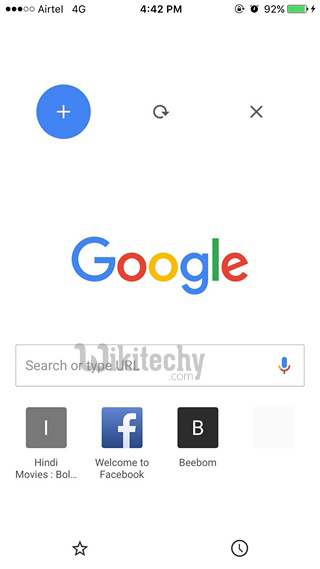A mobile screenshot of a Google search page, currently captured at 4:42 p.m. on an Airtel 4G network, with a 92% battery life indicated by both the battery icon and a lightning bolt, signifying it is charging. The status bar also includes icons for orientation lock and active alarm. The screen has a white background with dark gray text, adhering to Google's typical color scheme.

At the top center, there is a blue circle with a plus (+) icon, followed by a circular refresh arrow, and an 'X' button to close or clear tasks. Below that sits the prominent Google logo above the search bar, which contains a placeholder text saying "search or type URL" and to the right, a multicolored microphone icon for voice dictation.

Beneath the search bar are icons for frequently visited sites: one labeled "Hindi movies" with a partially visible “Bollywood”, and another for Facebook, titled "Welcome to Facebook". Each of these icons corresponds to a letter; 'I' for Hindi movies and 'B' for Facebook. Additionally, there are star and clock icons, likely for bookmarks and recent activity. The overall design remains minimalistic, typical of a standard Google search page.